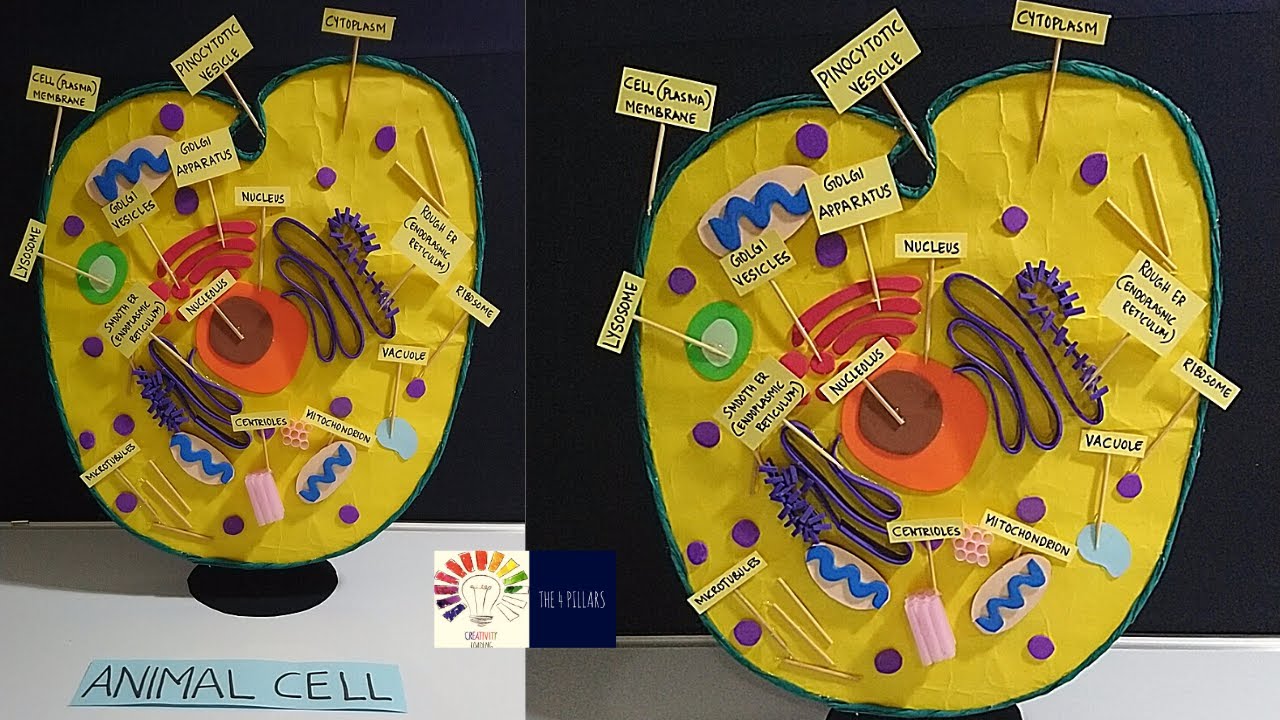The photograph features a detailed 3D model of an animal cell, likely a student's project, made using paper, construction paper, and possibly styrofoam, distinguished by vibrant colors for clarity. The model presents a cross-sectional view of the cell, highlighting essential components such as the nucleus, Golgi apparatus, lysosomes, and plasma membrane. These elements are meticulously labeled with toothpicks and small rectangular labels. The display comprises two images: the left photo shows the model in its entirety, sitting on an off-white base against a black background, possibly a blackboard, with a prominent card below it labeled "Animal Cell." This image includes the broader setup, while the right photo offers a detailed close-up of the model, omitting the background and base. The model features a green outer membrane, and orange, purple, red, and green parts representing various cell structures, all set against a yellow background where vacant spaces are filled.